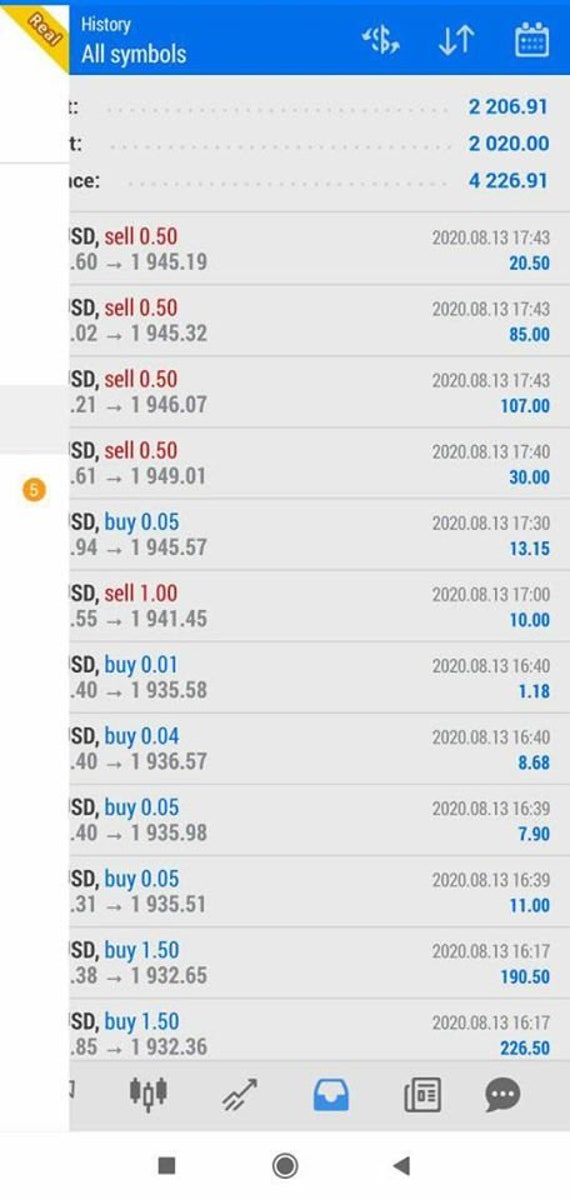This is a detailed screenshot of an app in portrait mode, prominently displaying a history section labeled "All Symbols" at the top. The topmost region features three icons: a money symbol with arrows, an up and down arrow, and a calendar icon. 

Beneath this, a diagonal yellow ribbon is shown partially displaying text, suggesting some information is cut off. The visible text reads "2,206.91" and "$2,020," hinting at possible financial data or transaction amounts. 

Further down, there are upwards of ten rows filled with text and numbers. Each row includes a date and a blue number on the right side, possibly indicating specific values or metrics. Additionally, these rows feature gray numbers transitioning via an arrow to another number, indicating some form of numerical transformation or conversion.

At the bottom of the screen, icons for various menu options are evident, including those for files, speech bubbles, and a newspaper. These likely represent different functional sections within the app.